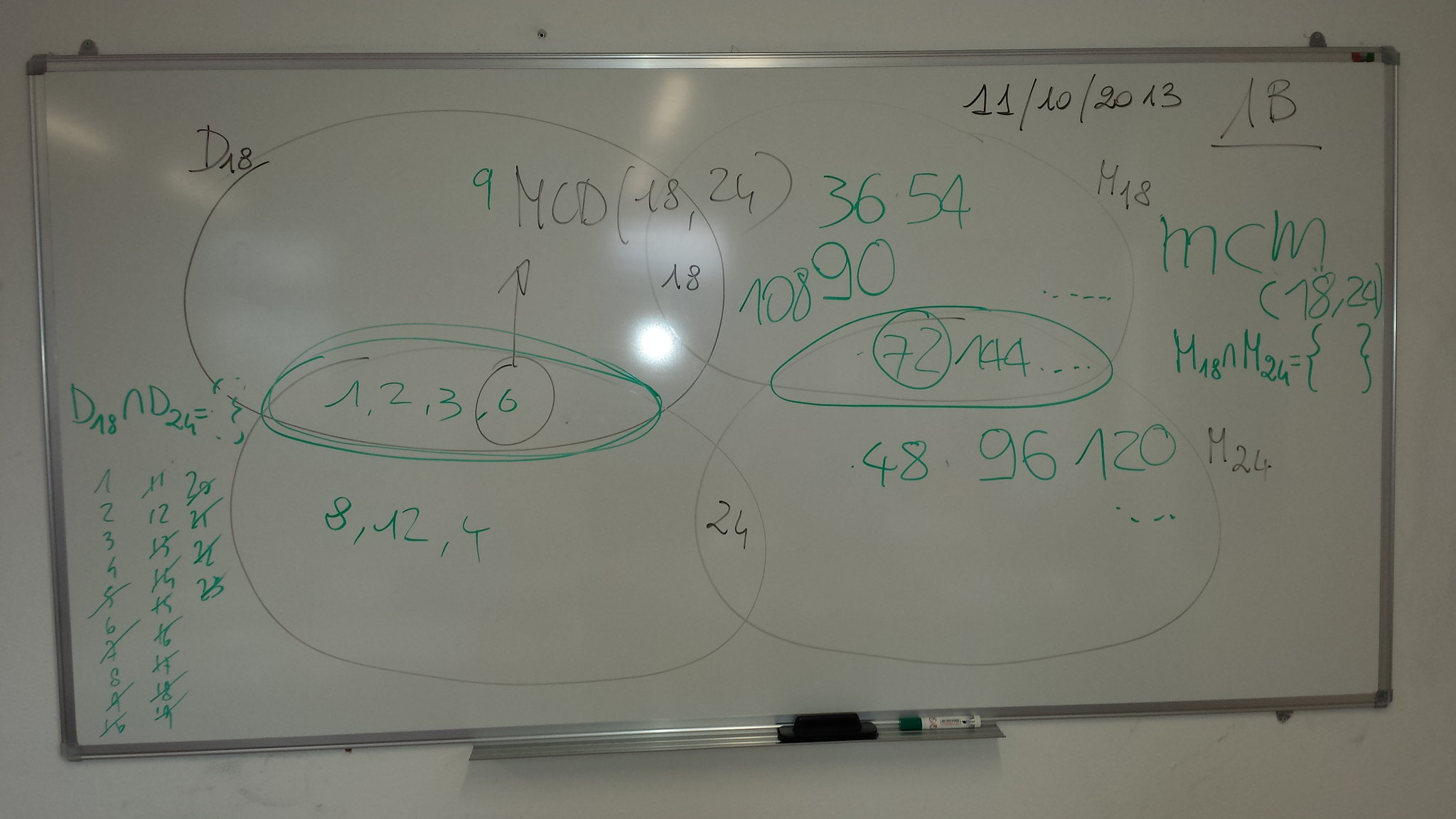Close-up of a rectangular whiteboard mounted on a white wall. The whiteboard, which is long and wide, features a collection of numbers, drawings, and illustrations, indicative of a mathematics lesson. In the upper right corner, the date "11-10-2013" is written in black marker. The whiteboard is a blend of green and black marker ink, displaying a series of complex figures and numerical sequences. Most prominently, four large intersecting circles dominate the lower portion of the board, forming a detailed Venn diagram. This intricate illustration suggests an attempt to explain a mathematical concept, possibly related to set theory, in a classroom setting.